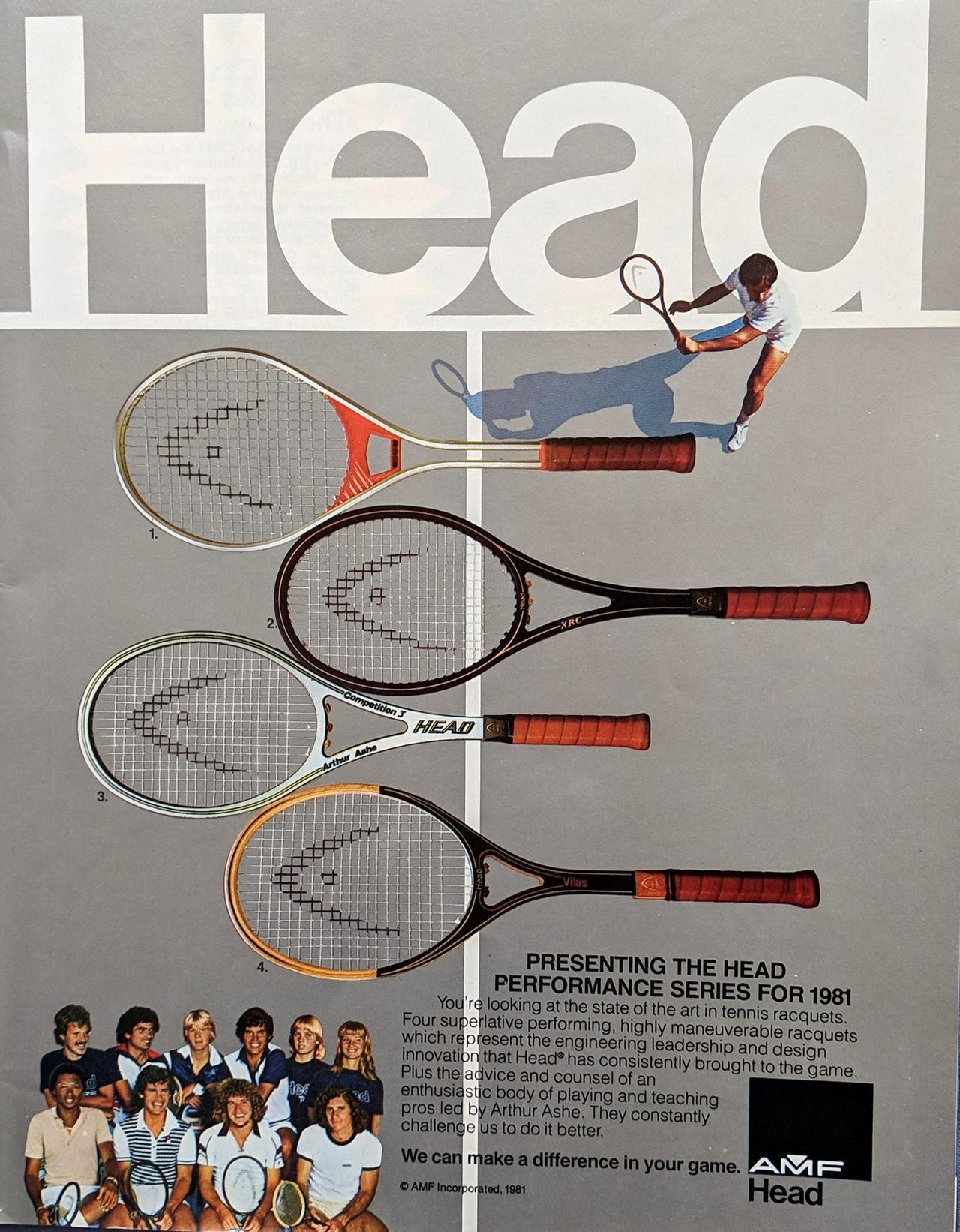The image is a full-color, digitally created promotional advertisement for HEAD. Dominating the upper part of the image, in large white letters against a light gray tennis court background with distinct white lines, is the word "HEAD." Below the heading, a man dressed entirely in white is captured mid-swing with a tennis racket, casting a shadow on the gray court. His presence is slightly upper right of the center. Centrally placed within the image are four colorful tennis rackets with the HEAD brand prominently displayed. In the lower left corner, a group of young, smiling people are holding tennis rackets, indicative of their enthusiasm and engagement. Directly opposite, in the lower right corner, is the AMF HEAD logo, providing official branding. Beneath the central elements, text introduces the head performance series for 1981, highlighting state-of-the-art, highly maneuverable rackets that represent advanced engineering and design innovation, supported by tennis pros led by Arthur Ashe. The advertisement emphasizes HEAD's commitment to enhancing players' game performance.